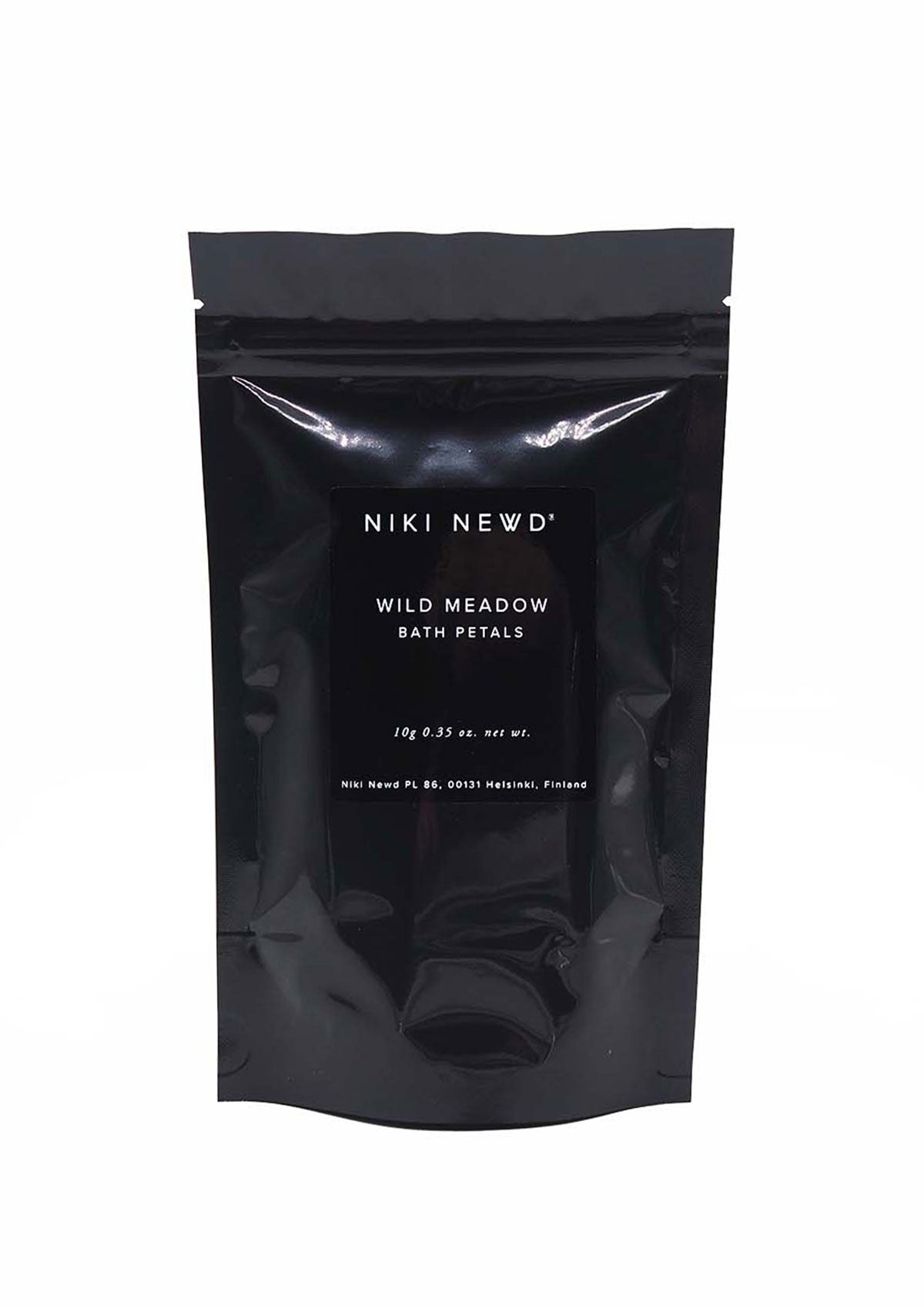The image displays a product set against a white background. The focal point of the image is a black, resealable vacuum seal bag made of reflective or shiny black plastic with a matte finish at the tear-off top. The bag features two notches on either side near the top, which allow for easy tearing to access the contents, and includes a resealable zipper inside. The label in the center of the packaging is also black with white text. The brand name on the label is "Niki Nude," spelled as N-I-K-I N-E-W-D. The product is identified as "Wild Meadow Bath Petals" and the net weight is specified as 10 grams (0.35 ounces). Additionally, a small address is visible at the bottom of the label: "PL86, 00131 Helsinki, Finland."